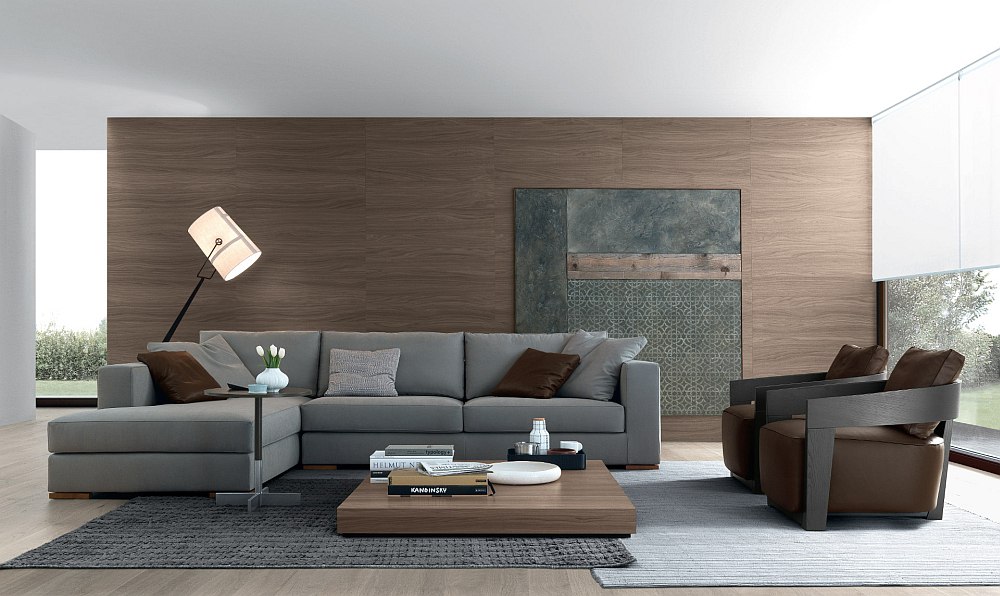This image features a modern living room that is both minimalistic and stylishly staged. The focal point is a large, L-shaped sectional sofa in a medium gray color, adorned with brown and light gray pillows, positioned in the bottom left-hand corner of the room. In front of the sofa is a low, legless, tan wood coffee table, measuring approximately four feet by four feet, and decorated with various accessories like books. To the right side, there are two brown recliner-style chairs with wooden arms and rounded backs. The background reveals floor-to-ceiling windows on either side, suggesting an open and airy atmosphere. Additionally, there is a wooden wall with a significant abstract art piece constructed from stone and wood behind the sofa, adding a touch of artistic flair to the room. The flooring includes sections of carpet that define separate areas for the furniture, enhancing the room's design. A large one-piece window shade is partially drawn, indicating a thoughtful approach to natural light management within this sleek, modern living space.